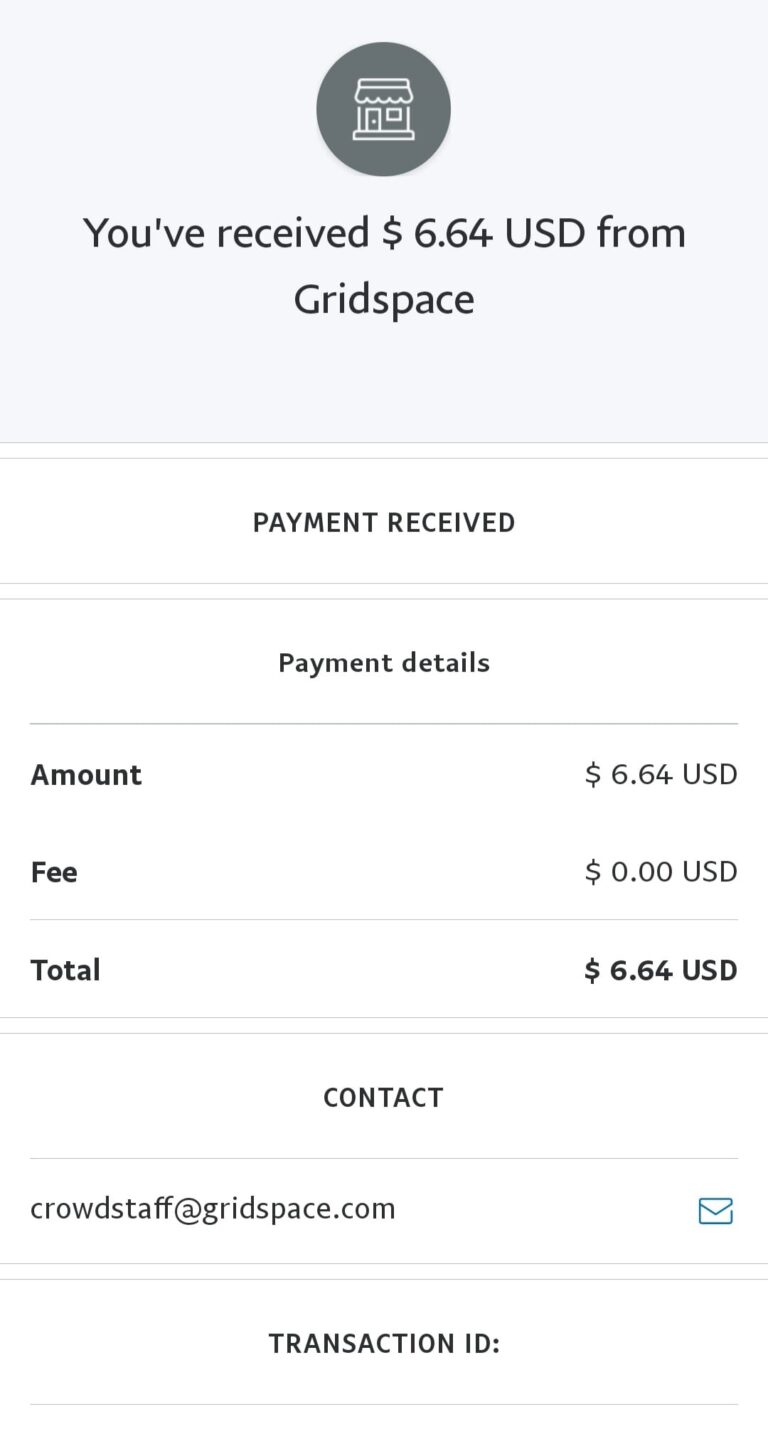This is a detailed screenshot of a mobile application displaying a recent transaction. At the top of the screen, there's a light gray rectangular banner with a dark gray circle centered at the top, featuring a white generic shop icon. Below this, a centered line of black text reads: "You've received $6.44 USD from". Beneath this message, there are two thin light gray lines separated by a white horizontal bar.

The main body of the page has a white background. In the center, bold black text in all caps states: "PAYMENT RECEIVED". Another pair of thin light gray lines separated by a white bar appears below this announcement.

Further down, bold black text that is not in all caps reads: "Payment Details". A medium gray thin line follows, leading to two rows of information. On the left, bolded black text reads: "Amount" and "Fee", and on the right, corresponding medium gray text states: "$6.44 USD" and "$0.00 USD" respectively. Below this, a thin light gray line appears.

Next, in the left column, bold black text reads: "Total", with the amount, "$6.44 USD", bolded and aligned to the right. Another set of thin light gray lines follows.

Centered beneath this, medium gray text in all caps reads: "CONTACT". Another thin light gray line follows. Finally, justified to the left, small black text reads: "crowdstaff@gridspace.com", with a blue envelope icon aligned to the far right.